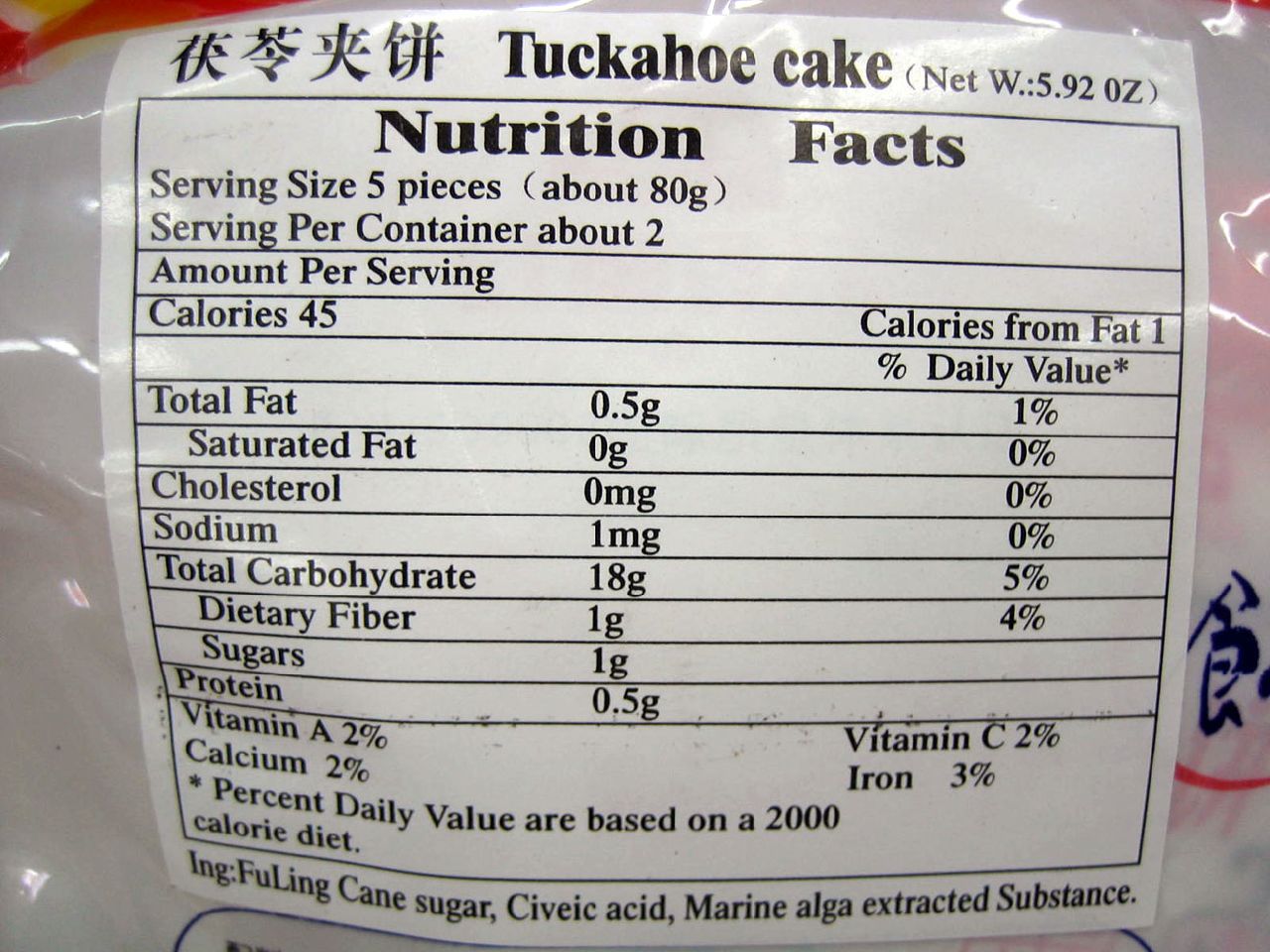The image is a digital photo showcasing the backside of a white package. The central focus is a white square label with "Nutrition Facts" prominently displayed in bold black letters. The upper part of the label starts with a section in a foreign language, likely Chinese or Japanese, followed by English text. It indicates "Tuckahoe Cake, Net Wt: 5.92 oz". Below this, detailed nutritional information is provided for a serving size of five pieces (approximately 80 grams), with around two servings per container. The label lists per serving: 45 calories (one calorie from fat), total fat 0.5 grams (1% daily value), 0 grams of saturated fat (0%), 0 milligrams of cholesterol (0%), 1 milligram of sodium (0%), 18 grams of total carbohydrates (5%), 1 gram of dietary fiber (4%), 1 gram of sugars, and 0.5 grams of protein. Additional nutrient details include Vitamin A, Vitamin C, calcium, and iron, all specified with their respective daily values. Ingredients listed include fuling, cane sugar, citric acid, and marine algae extract. The label concludes with a note that the percent daily values are based on a 2,000-calorie diet. The package itself is partially visible, showing some indistinguishable patterns or texts.